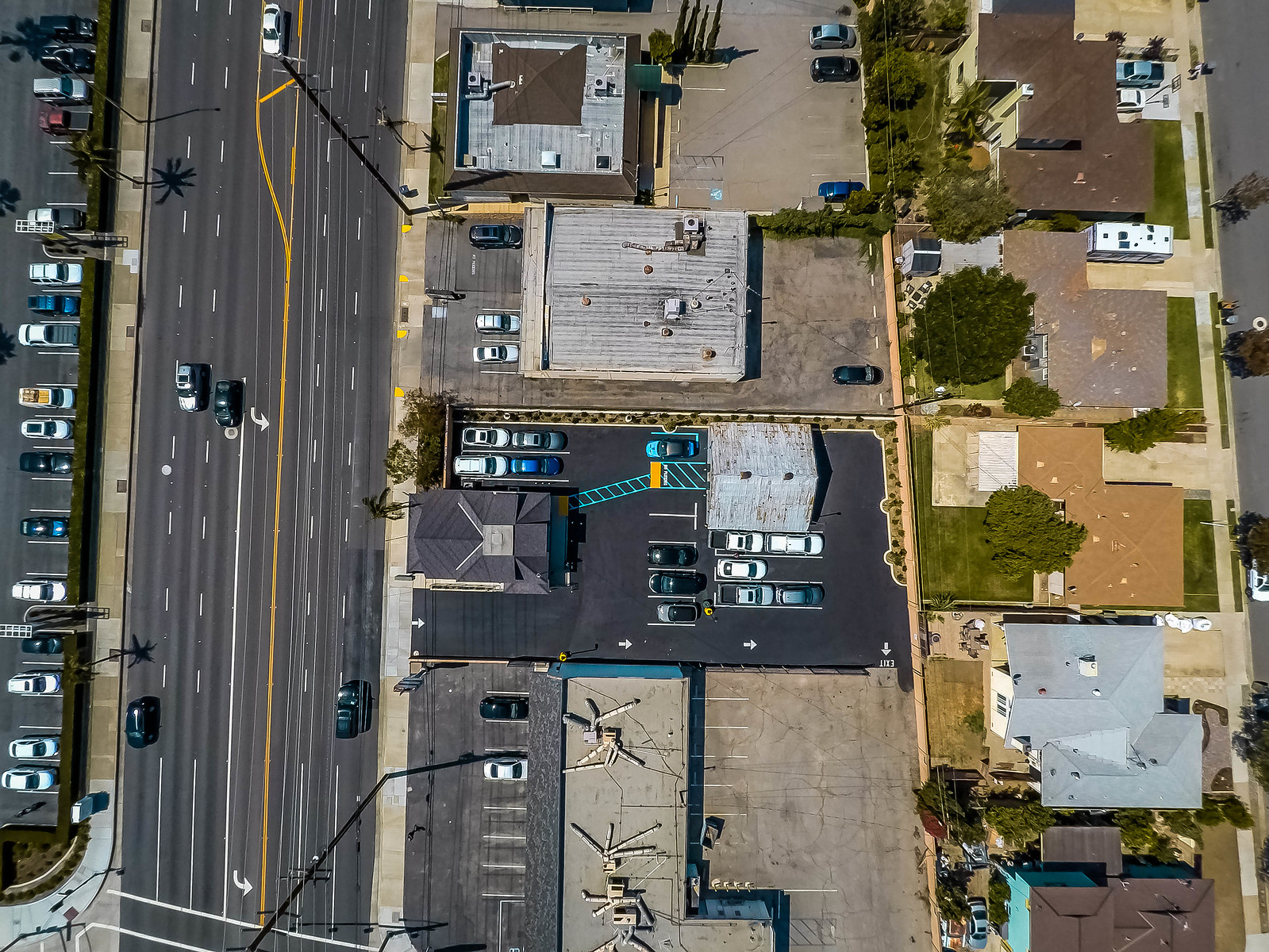Aerial View of Urban Landscape: On the far left, a neatly organized parking lot is visible, with clear markings delineating the parking spaces. Most of these spaces are occupied by vehicles, with just a few remaining open. Adjacent to the parking lot and extending horizontally across the image is a broad six-lane highway, bustling with traffic. To the right of the highway, the tops of several buildings come into view, characterized by their varied architectural designs. Further to the right, a residential neighborhood emerges, revealing a collection of homes with distinct features. Some driveways have cars parked, while others are empty. The house at the top of this section includes a basketball hoop in its driveway, followed by another home with a camper parked in front. The subsequent houses do not have any vehicles in their driveways. Each home is supplemented with trees in their backyards, adding a touch of greenery to the scene. Additionally, a few pedestrians can be spotted walking on the sidewalk that runs in front of the homes.